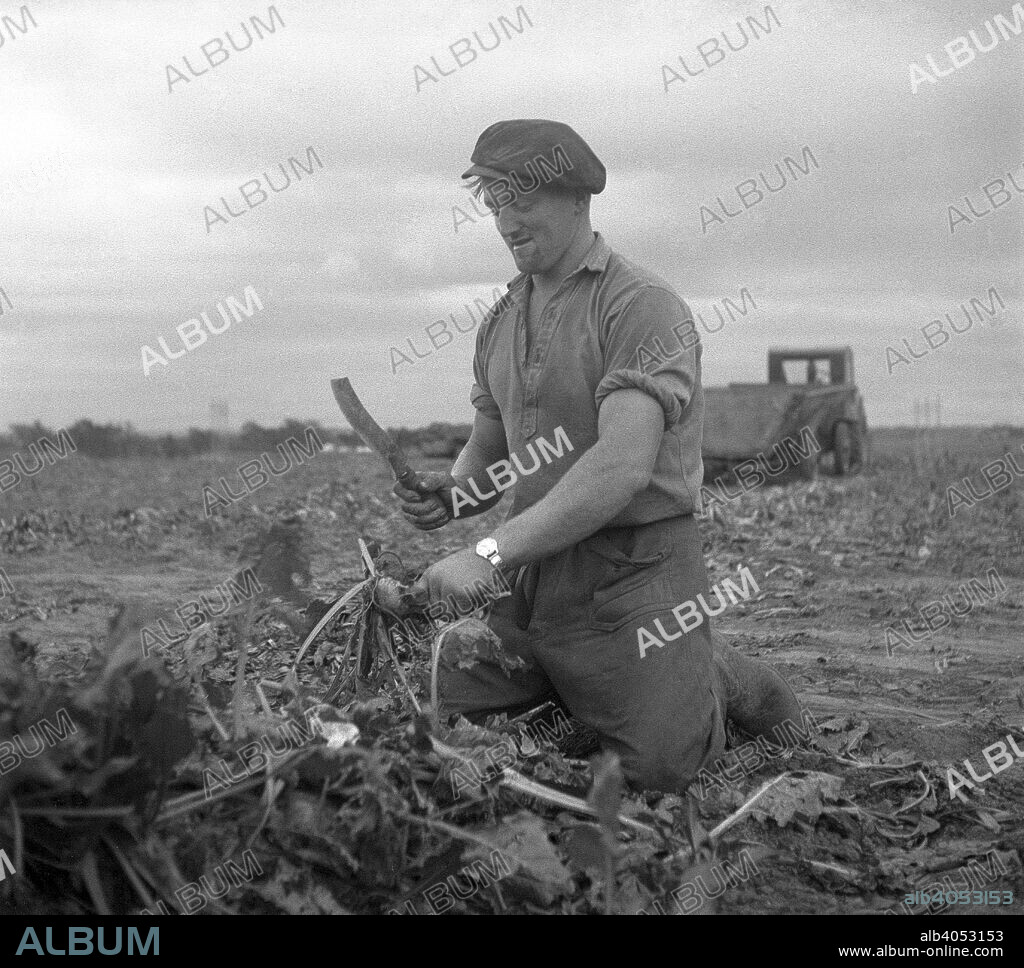This is a large, square, black and white photograph with the word "ALBUM" diagonally overlaid in white and gray all caps throughout the background, resembling a stock photo watermark. At the bottom is a black rectangular border, with "ALBUM" in blue on the left and "ALB4053153" along with "www.album-online.com" in white on the right. The image captures a vintage scene of a Caucasian farmer in a field. He is kneeling and appears focused as he readies to cut a vegetable—likely a beet—with a knife in his right hand. The farmer, who has a smile on his face and a light beard, is wearing a cap that resembles a plaid beret, a button-down shirt with rolled-up sleeves, dark pants, and boots. He sports a watch on his left wrist. Behind him, slightly blurry, is agricultural machinery, possibly a tractor with a trailer or a combine. The background reveals a harvested field with scattered stalks, an overcast sky, and a distant tree line, giving the whole scene a hardworking, rustic charm.